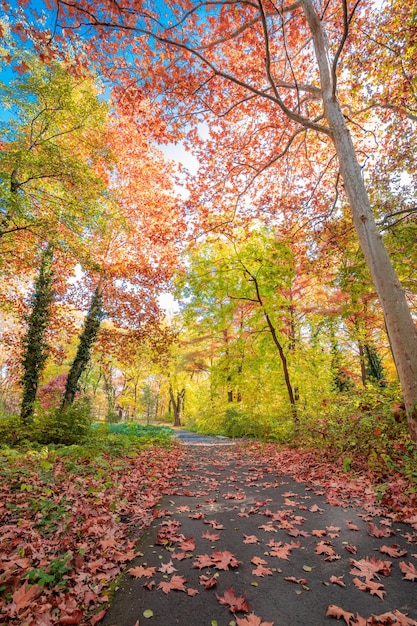This detailed photograph captures a serene autumn scene in a forest featuring a narrow asphalt pathway, covered abundantly with brown and red-orange leaves. The road, appearing as a dark, gray asphalt, winds deeper into the woods, flanked on both sides by ground similarly blanketed with autumn leaves. The forest canopy showcases a vibrant tapestry of seasonal colors, with trees predominantly exhibiting various shades of orange, brown, and yellow-green. One prominent tree on the right has striking brownish-orange leaves, while others display a mix of light greenish-yellow and bright orange foliage. The bright blue sky peeks through the gaps between the tall trees, adding a splash of crispness to the cool, sunny autumn day. Further along the path, there is more foliage and climbing vines clinging to the trunks, creating a picturesque atmosphere as the road stretches forward into the heart of the colorful woodland.